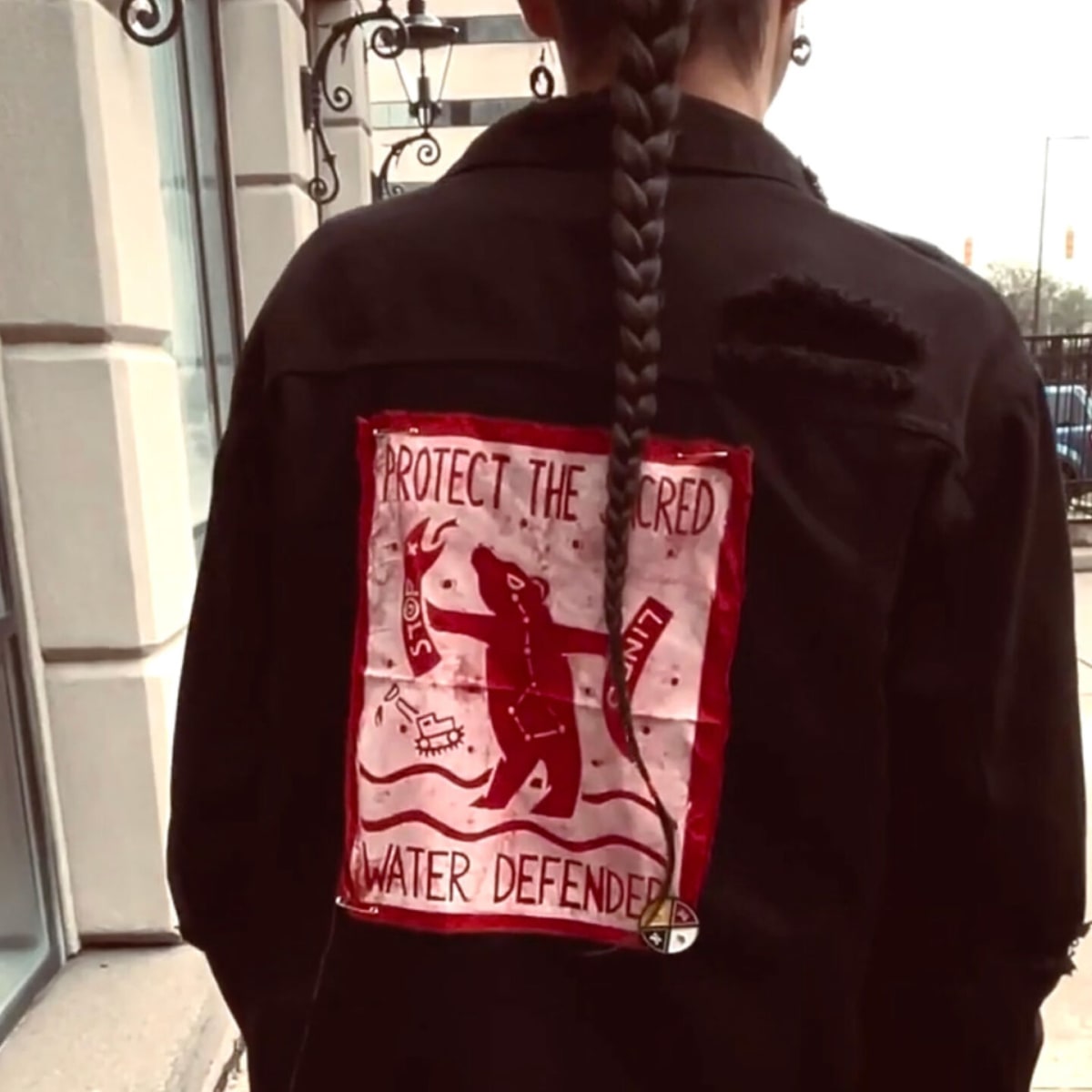The outdoor image captures a woman seen from behind, standing against a backdrop featuring a large white brick building with metal streetlights, a distant SUV, trees, and a metal fence. Her dark brown hair is intricately braided into a long ponytail that extends down her back. She's wearing a black jacket with a noticeable hole on the top right side and sportsey earrings. The jacket has a pinned artwork design centered on the back, bordered in red and secured with safety pins on three sides. The design displays the text "Protect the Sacred Water Defender" in red and white. The braid partially obscures some letters and details, but visible imagery includes a figure holding two signs, with the legible sign saying "Stop." The image, though slightly blurry, clearly shows the bright daylight setting.